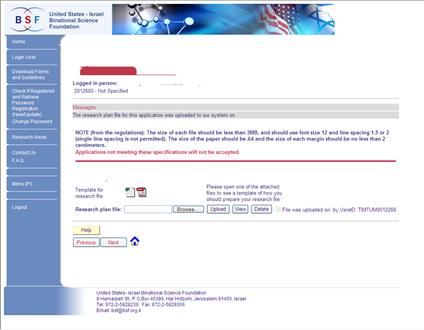**Detailed Caption:**

The image captures a screenshot of a website page, primarily landscape in orientation and nearly square in shape. The photo features a thin black border along the left side and top, but none on the bottom or right. The webpage is set against a predominantly white background, with various colors accentuating different sections.

At the top-left corner, there is a long rectangular box containing blue font. Next to it is a logo that reads "BSF," where 'B' is in blue, 'S' in red, and 'F' in light blue. This logo is accompanied by two interconnecting circles, missing their centers and sides. Below the logo, text reads "United States Environmental Science Foundation," accompanied by a secondary logo. The secondary logo appears to feature the United States flag in the background, possibly incorporating an Israeli star and other scientific icons.

A vertical blue border runs along the left side of the page, with white font and clickable boxes for navigation.

The central portion of the image predominantly displays a white background. At the top, there is a red tab, followed by some text in a bluish-purple font. Below this text are two thin, long gray boxes spanning horizontally across the screen, containing purple font. These are followed by additional text boxed in red with a red border running horizontally.

Notably, there is a "browse" box on the page, suggesting that the website might be older in design. The overall aesthetic reflects a vintage web layout characterized by distinct sections and colorful borders.